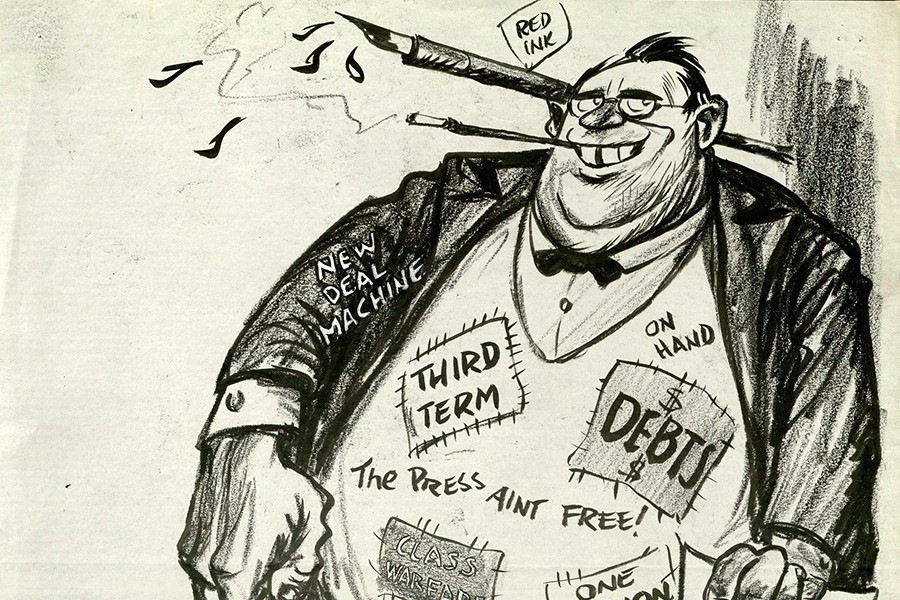In this detailed black and white satirical cartoon, we see a very heavy, chubby man with short hair, wearing glasses and a double chin, giving him a rather devious appearance. He is wearing a slightly ill-fitting black coat over a white vest adorned with numerous inscriptions. Prominent among them are "Third Term," "On Hand," "Debts," "The Press Ain't Free," "New Deal Machine," and other phrases hinting at financial and political themes such as a money symbol and possibly "Class, War." 

A long cigarette attached to a stick is perched in his mouth, emitting smoke, further adding to his caricatured villainy. Behind his ear is a large pen dripping with ink, labeled "Red Ink," which appears to be staining the paper, symbolizing fiscal irresponsibility. The setting suggests political commentary, possibly portraying the large man as a dubious candidate for a third term in office, as hinted by the phrase "Third Term" emblazoned across his vest. His overall demeanor, with a shifty smile and shaded nose, indicates he's up to no good, highlighting the cartoon's satirical message.